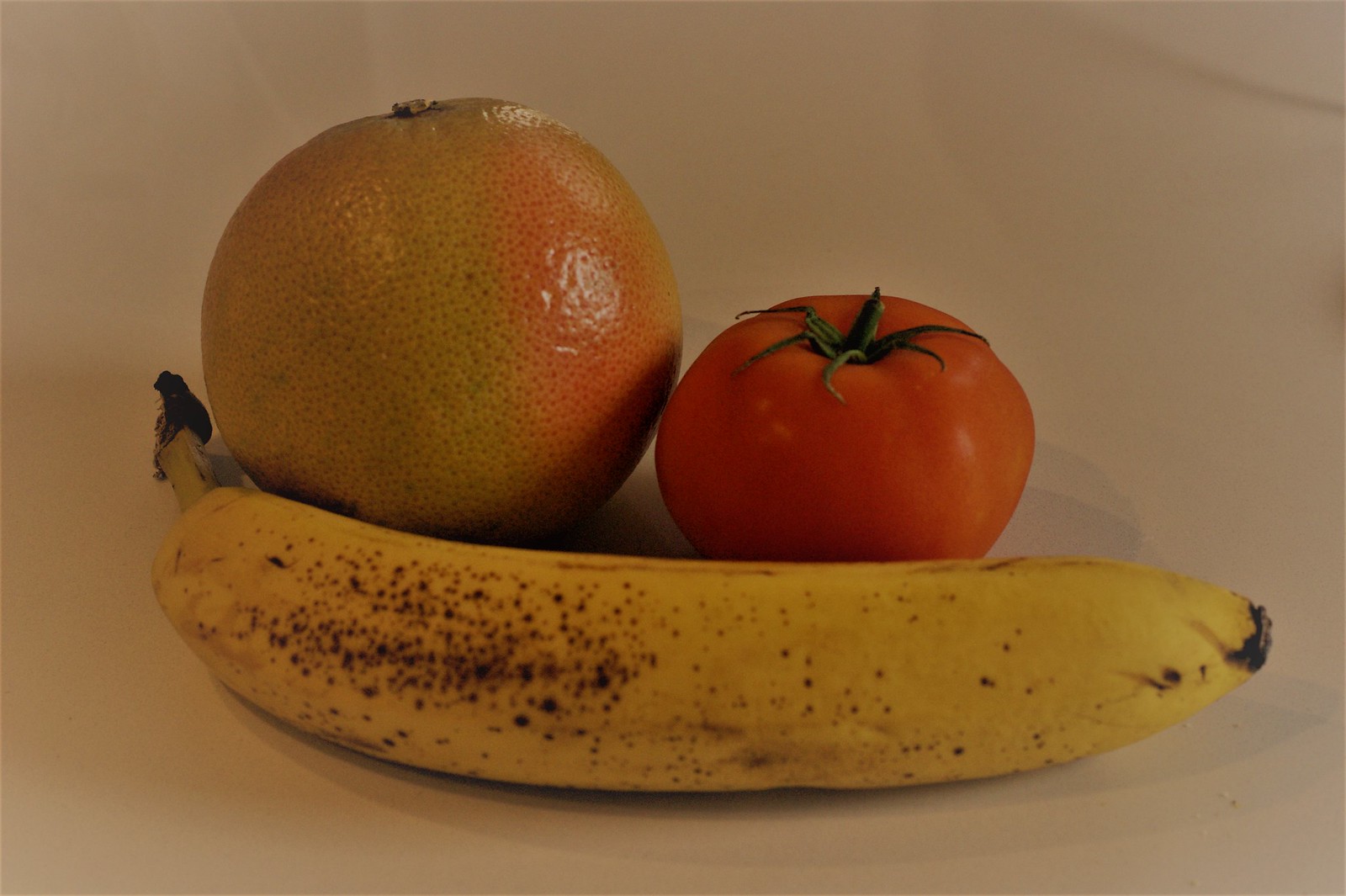In this image, three distinct pieces of fruit are displayed with notable details. In the foreground, an overly ripe banana, speckled with numerous brown spots, lies horizontally from one end to the other, indicating it’s likely past its ripeness. Just above and to the left of the banana is a uniquely colored grapefruit. The majority of its rind is a pale green hue, transitioning to a reddish-pink tint on the right side, creating a captivating color gradient. Positioned to the right above the banana, a vibrant red tomato, approximately half the size of the grapefruit, features a cluster of six green leaves sprouting from its top, adding a fresh contrast. The composition highlights the varied textures, colors, and states of ripeness of the fruits, creating an intriguing visual tableau.